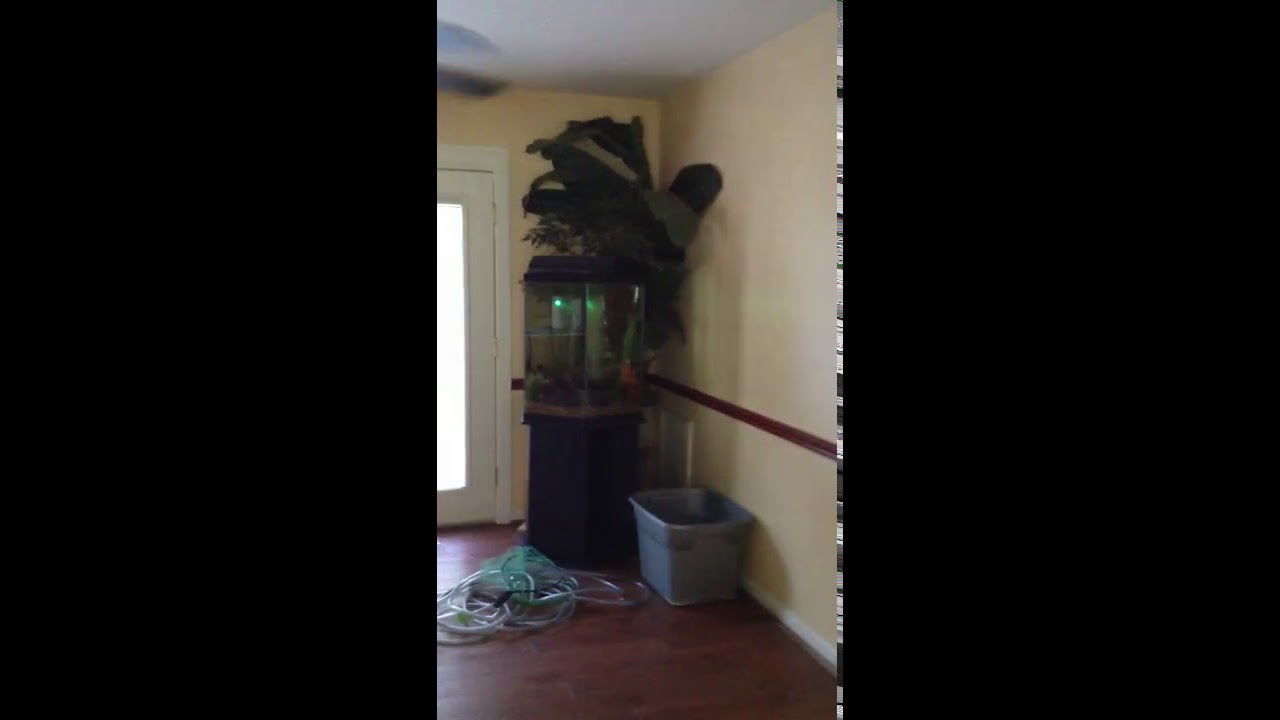The image captures a corner of a room featuring a freestanding rectangular fish tank with a black pedestal. The tank is filled with water, rocks along the bottom, and possibly some plants inside. The glass tank is illuminated by a small light. Behind the tank is a large green tropical plant adding a touch of natural green to the scene. In front of the tank, there are some fish tank accessories including a tangled pile of plastic tubes and cables, as well as a rounded square blue Tupperware bin. The room boasts dark wooden flooring, magnolia beige walls with a brown piece of molding running horizontally halfway up the wall, and a white ceiling with a ceiling fan. The tank and accessories are situated near a white door with a long rectangular window pane.